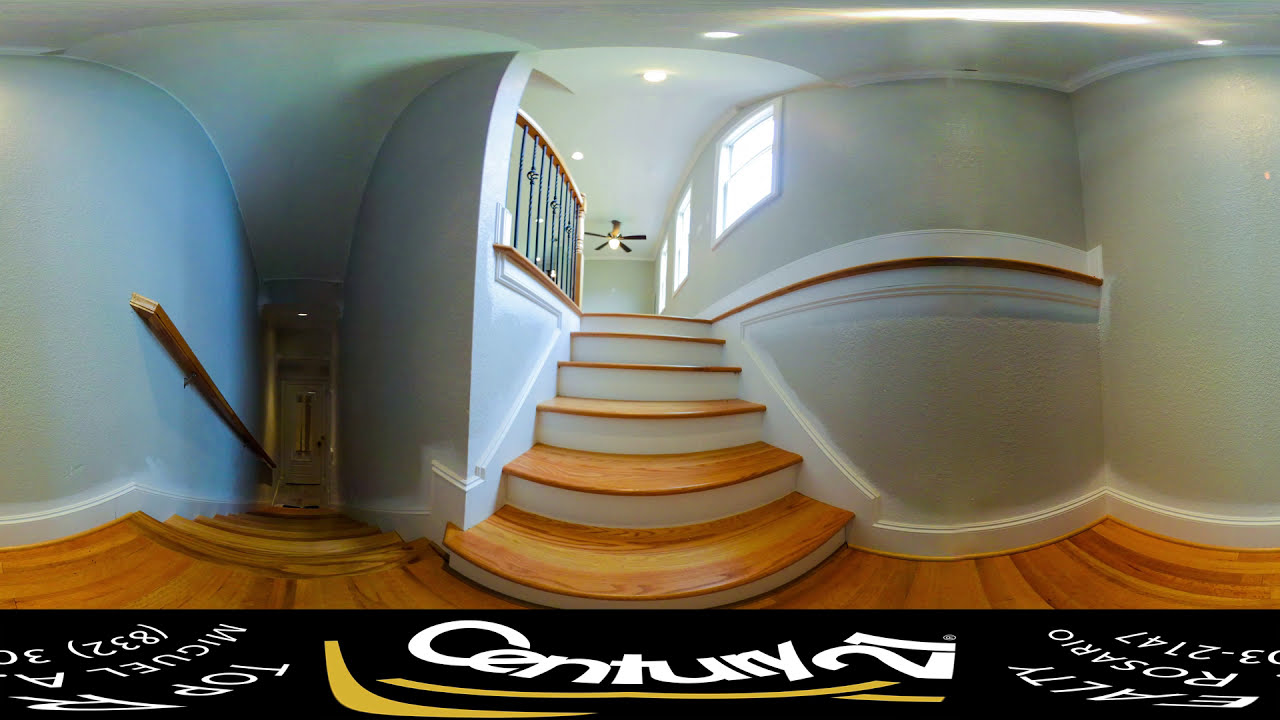The image appears to be an altered real estate advertisement for Century 21, featuring a distorted photograph of an empty house interior. At the center of the image is a short stairwell with six or seven steps, leading to an upper floor. The steps have wooden treads and white-painted risers, complemented by a wooden railing with black fittings on the left side. The flooring throughout the house is wooden, with a brown hue tinged with yellow. The walls are crisp white, and there are three windows on the upper level, allowing in natural light. A ceiling fan with an attached light bulb is mounted above the stairs, illuminating the scene. Distorted text at the bottom of the image, set against a black background, bears the Century 21 logo underscored by yellow lines. Additional text includes contact details and the real estate agent's name, although the unusual, topsy-turvy font makes it difficult to decipher. This manipulated image likely highlights the distorted nature of the marketing materials, compromising the clarity of the advertisement.